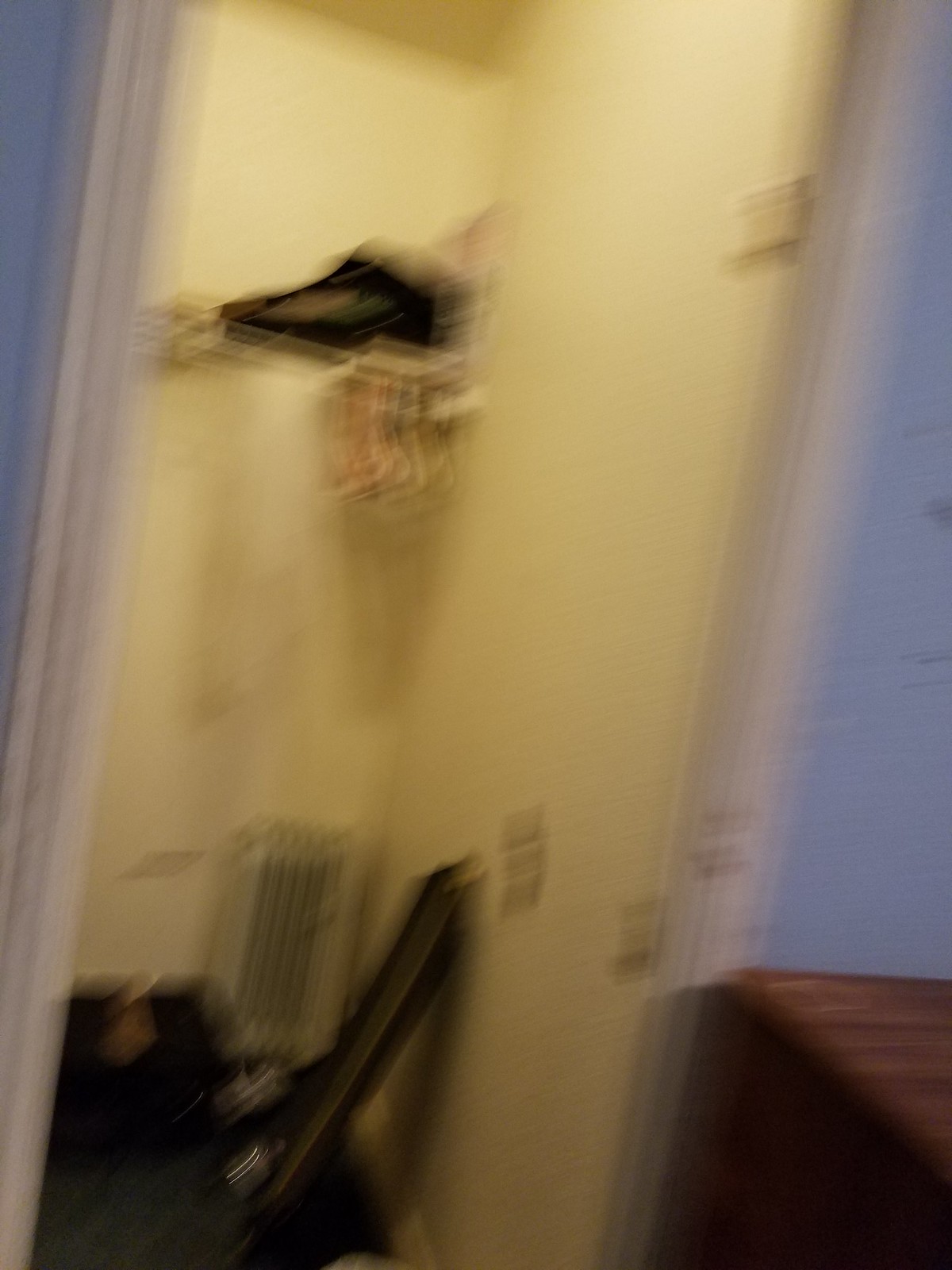The digital photo captures a dimly lit, blurry interior scene, with noticeable motion blur and a tilt to the right. The image showcases a closet or entryway bathed in yellowish light, likely from an old incandescent bulb. The closet, which lacks a door, features white walls and a wire shelf at the top adorned with plastic hangers and a black object, possibly a bag. A cream-colored portable electric space heater is positioned on the floor, flanked by another black item, shapely like a guitar case. To the right, inside the open doorway, a brown wooden trunk is visible. The surrounding area includes a mixture of light blue and purple walls, adding a subtle contrast to the scene. The floor appears cluttered with indistinct piles of black items, adding to the untidy appearance. Overall, the photo is very blurry, making it difficult to discern finer details.